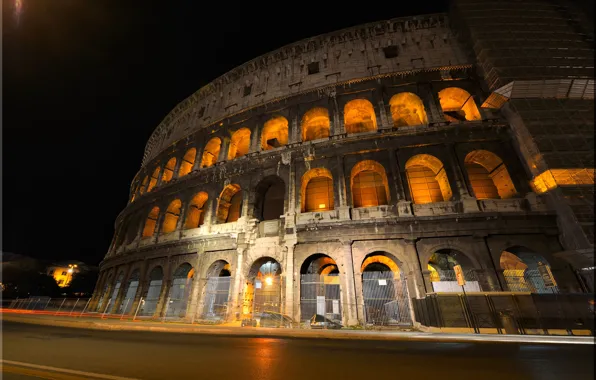This nighttime photograph captures a grand, Colosseum-like structure, possibly the Roman Colosseum. The monumental, rounded building, characterized by its three stories of arches, stands imposingly close to a street, separated only by a chain-link fence. Each arch glows warmly with amber or golden light, creating a striking contrast against the night sky. The upper two levels of the structure are particularly illuminated, while the bottom level is less so, suggesting entry points or doorways that are dimmer. In the background on the left side, another faint golden light highlights an unclear, distant structure. The entire scene gives a vivid sense of both majesty and historical significance, enhanced by the subtle details of cement and metal present in the architecture. The picture, taken from street level, provides a comprehensive and intimate view of this ancient, storied edifice.